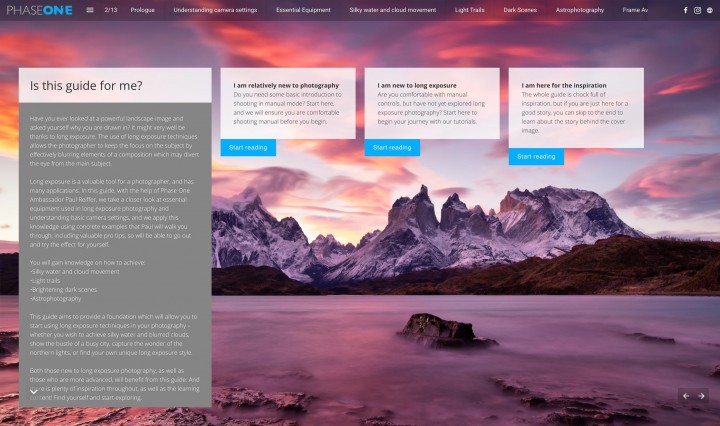Screenshot of Phase One's website: In the upper left corner, the "Phase" logo is displayed in a thin gray font, with "One" in a thicker blue font. On the right side, there is a bar that includes an element resembling "2/13." This bar extends horizontally across the screen, connecting various menu options. 

Following the "2/13" marker, the menu items include "Packages," "Understanding Camera Settings," "Essential Equipment," "Dark Services," and several other options. 

Beneath the menu bar, a vertical section labelled "Is This Guide For Me?" is situated. To its right are three boxes, each featuring a blue "Start Reading" button. The background image depicts a rugged, canyon-like terrain that evokes the surface of an alien planet.